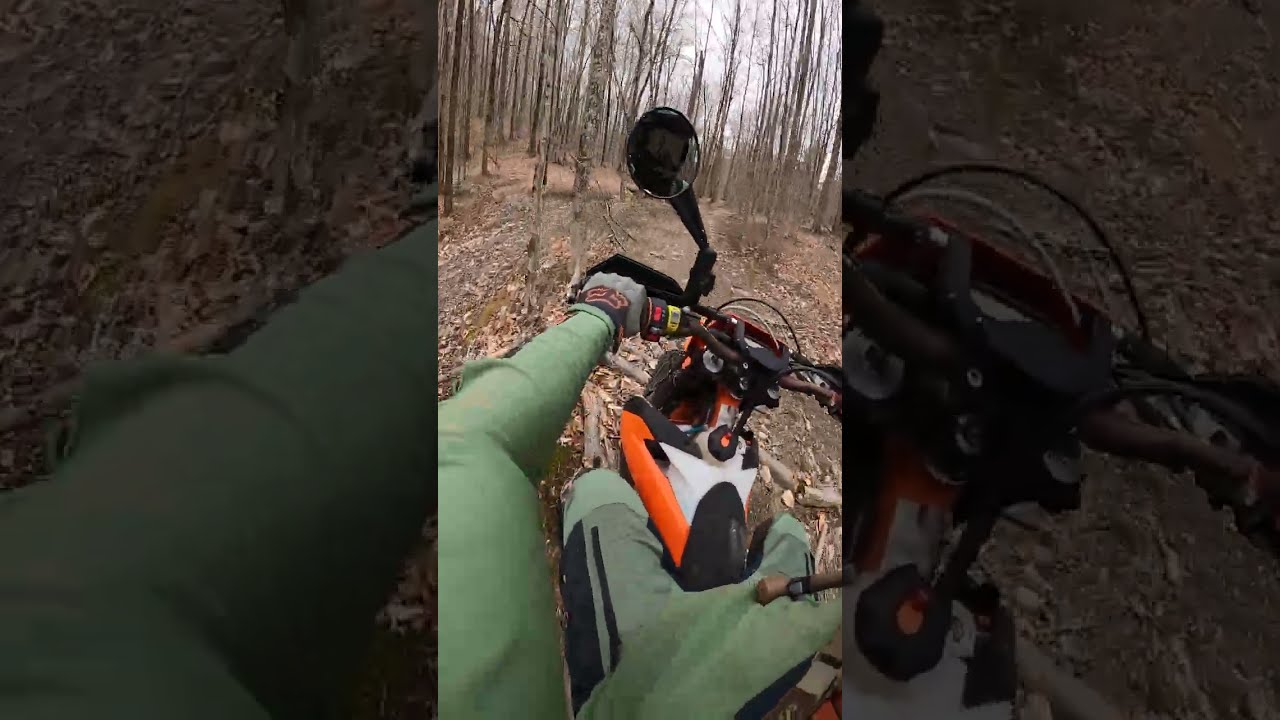The image is a detailed, first-person view from a GoPro camera mounted on a helmet of a motorcyclist riding through a desolate wooded area in the fall. The rider is piloting a grey, orange, and black motorbike along a dirt path blanketed with fallen leaves. Tall, bare trees with no foliage line the path, indicating the season is autumn. The sky overhead is an overcast greyish-blue, giving the scene a cold, quiet atmosphere. The motorcyclist is dressed in a green and black outfit, including a long-sleeved olive green top, matching green shorts or pants, and green Fox gloves. Their left hand grips the handlebar, and a rearview mirror is visible in the upper center of the image. The scene is captured in photographic representational realism, emphasizing the somber, tranquil mood of the fall day.